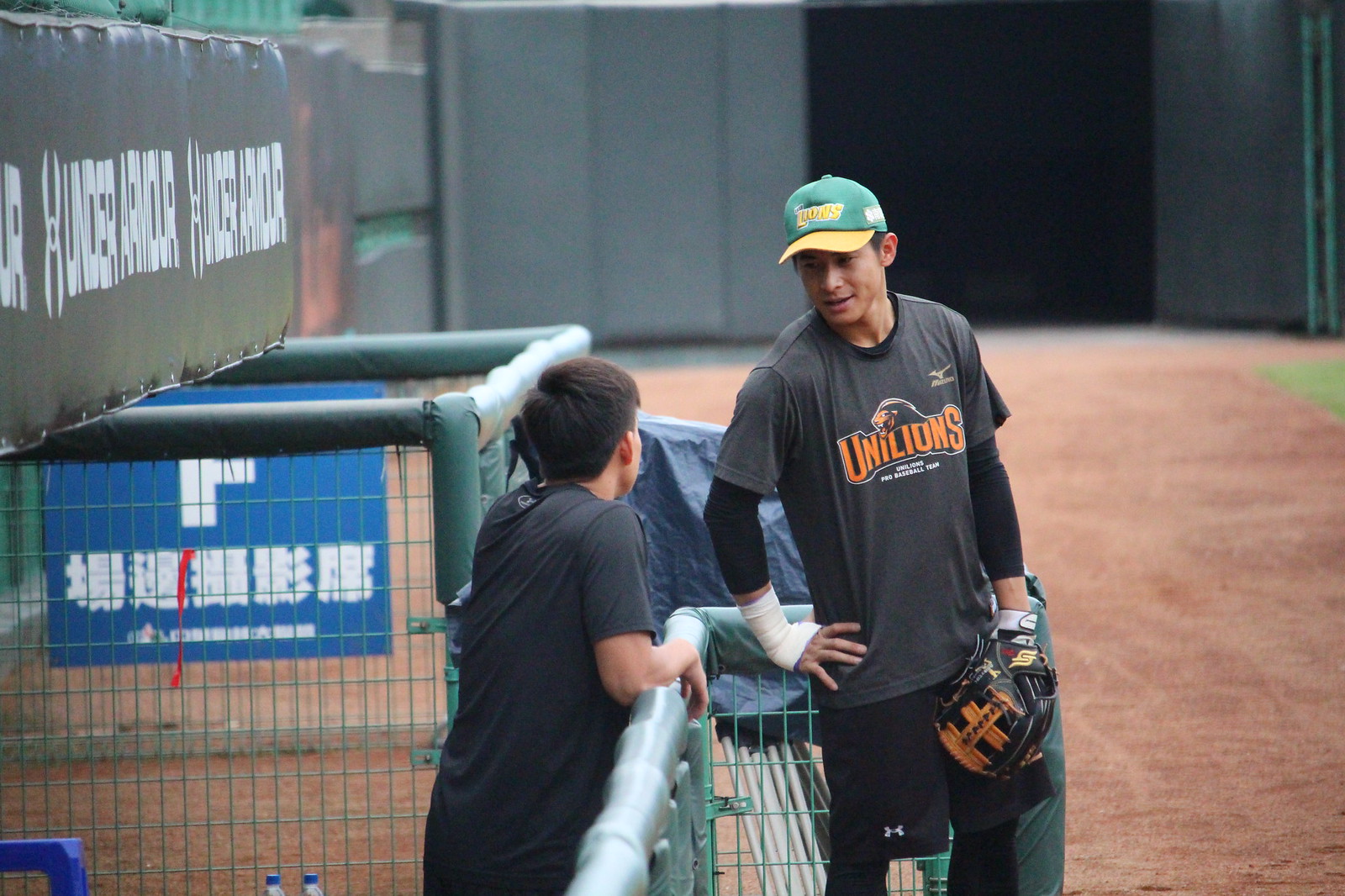In the photograph, we see two individuals, a baseball player and a younger fan, engaged in conversation near a green metal fence on a baseball diamond. The central figure is the baseball player, dressed in a distinctive uniform: a black t-shirt with "UniLions" written in orange, over a black long-sleeve shirt, black shorts, and black tights. He is sporting a green and yellow hat with "Lions" embroidered in yellow and has a brace on his right hand, which rests on his hip. His other hand holds a black and orange baseball glove. Beside him, leaning on the fence, is the young fan, whose short hair and dark shirt are visible from behind.

The scene is set against a backdrop of brown dirt and a grass infield with high walls on either side displaying text that is difficult to read, possibly in Asian script. A door behind the pair sits ajar, hinting at potential activity or movement within the facility. The overall setting suggests a practice environment, with the player appearing to be in preparation for a game. The green decor of the field and fencing adds a vivid contrast to the otherwise earthy tones of the infield.